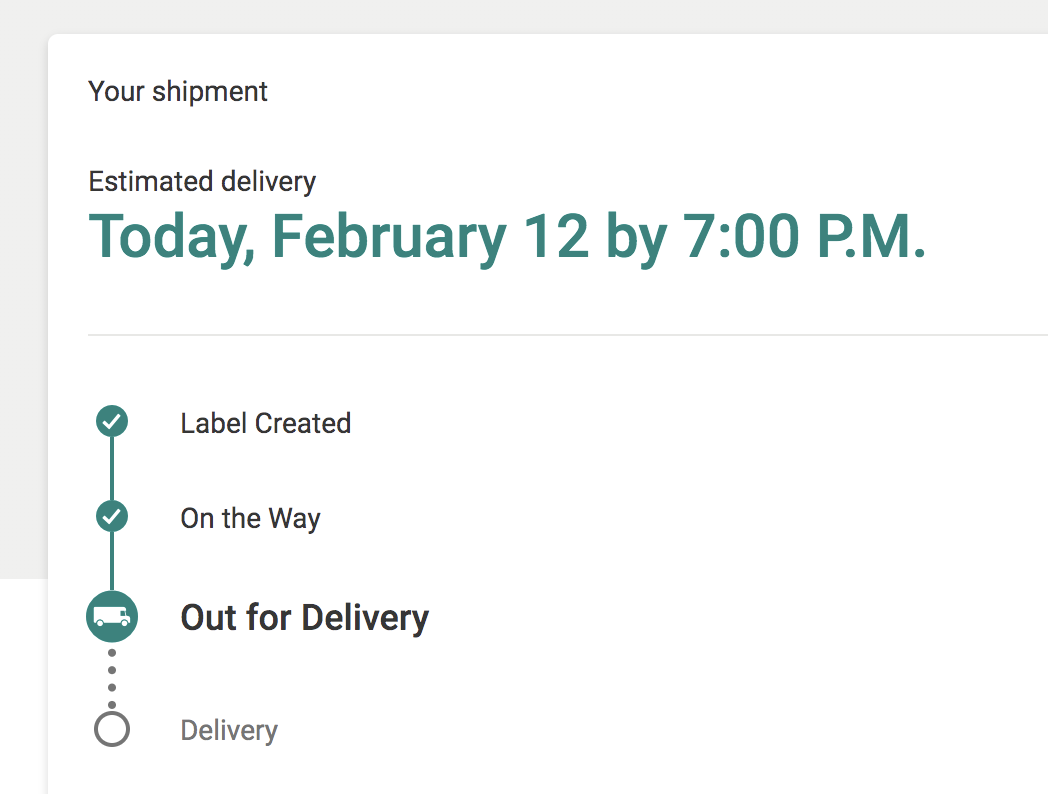This image features a detailed delivery status update with a clean and organized design. The border of the image is framed by a heavy light blue box, with an additional thin light blue line creating a double-border effect. Within this border is a white paper background. In the top-left corner, the text "Your shipment estimated delivery" is displayed, with "Today, February 12th by 7:00 p.m." highlighted in bold blue print below it.

Beneath this header, there is a horizontal thin blue line followed by a series of status indicators. The first indicator is a blue circle with a checkmark labeled "Label Created." A vertical line connects this circle to the next indicator, another blue circle with a checkmark, labeled "On the Way." The sequence continues with a third, larger blue circle featuring an icon of a delivery truck and the label "Out for Delivery," which is currently highlighted to denote the package is in this stage. Further down, there are four smaller dots leading to a final circle that reads "Delivered."

Overall, the visual elements suggest the package is actively out for delivery and scheduled to arrive by 7:00 p.m. on February 12th. The design is framed by consistent blue border lines, with the main content neatly organized within the box that starts about a quarter of the way up the left side and extends all the way around the top.